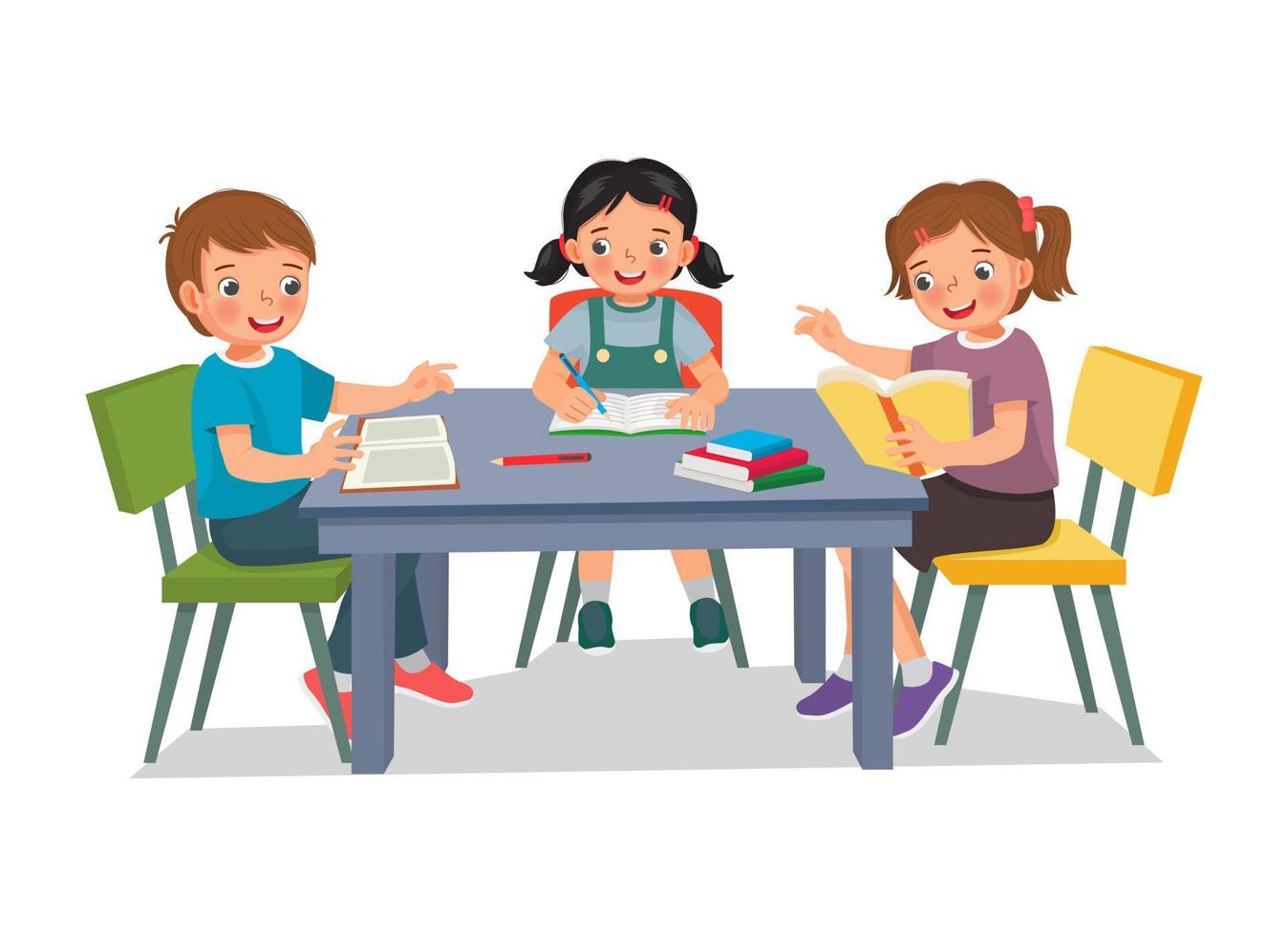The colorful cartoon image depicts three children with white skin, rosy cheeks, and cheerful expressions sitting around a gray table, engaged in reading and writing activities. Each child sits on a distinctively colored chair: the boy on the left is in a green chair, wearing blue pants, red shoes with white trim, and a light blue short-sleeved shirt. He has brown wispy hair and an open book in front of him, pointing towards the girl opposite him. The girl on the right, seated in a yellow chair, has brown hair tied in pigtails with pink ribbons, a purple short-sleeved t-shirt, and black pants. She appears to be reading from a yellow book with a red spine. In the middle, a girl with black hair in pigtails tied with red ribbons sits in a red chair. She is dressed in green overalls over a bluish-green shirt and blue shoes with white trim. She is diligently writing in an open book, possibly a notebook, using a blue pen or pencil. The table also holds additional books, suggesting a collaborative or study environment.